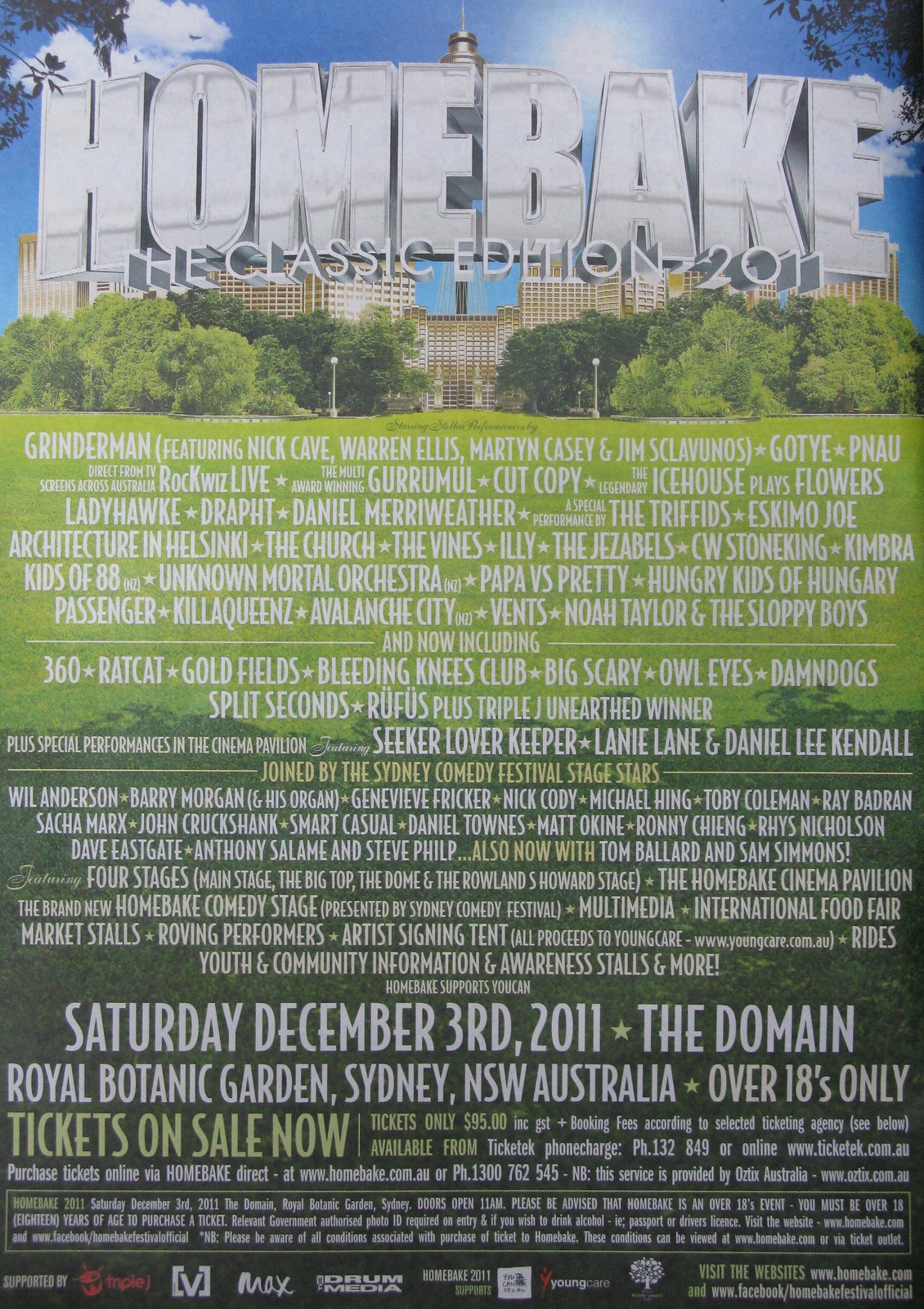The poster advertises a large music festival taking place at the Domain Royal Botanic Garden in Sydney, NSW, Australia, on Saturday, December 3, 2011. At the top of the poster, a grand, hotel-like building looms with large, silver lettering that reads "Home Bake: The Classic Edition 2011." This building is framed by lush green trees and a grassy expanse below. The grass area contains an extensive list of performers, including Nick Cave, Warren Ellis, Martin Casey, The Vines, Illy, The Jezebels, Gotye, Ladyhawke, Architecture in Helsinki, Cut Copy, Icehouse, Flowers, Eskimo Joe, and many more, indicating a densely packed music festival lineup. Below this, in bold letters, details about the event are provided: "Saturday, December 3, 2011, the Domain Royal Botanic Garden, Sydney, NSW, Australia, Over 18s only. Tickets on sale now." Additional information about ticket purchase is also included at the bottom.